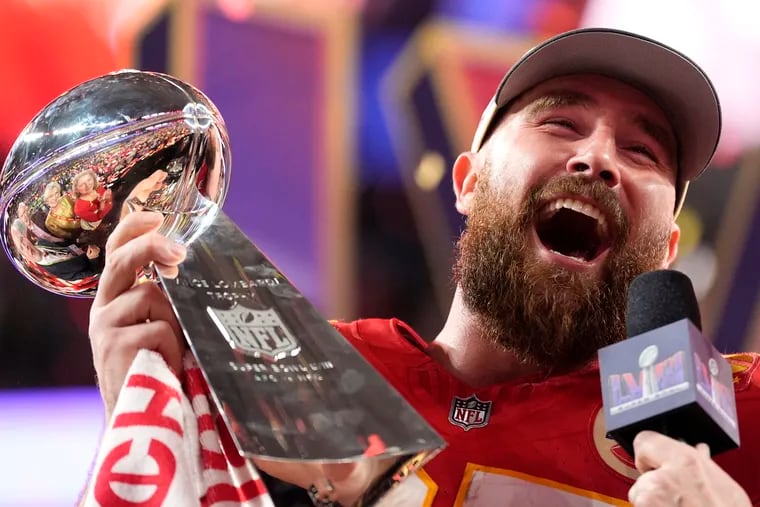This close-up photograph captures the jubilant moment of Travis Kelsey, an NFL athlete, holding a football championship trophy. He's beaming with joy, his mouth wide open in laughter. Kelsey sports a brown beard and very short hair, and is wearing a red Kansas City Chiefs jersey with white numbers outlined in gold. A beige-billed baseball cap rests on his head. The intricately detailed trophy he clutches features a silver football atop a flat silver plate, emblazoned with the NFL emblem. The sheen of the football reflects the surrounding crowd, adding layers to the celebratory atmosphere. In front of him, a microphone, identifiable by its black foam top and a square containing a "LIVE" insignia with a football trophy image, captures his excited reactions. The muted background radiates hues of purple, blue, and red, enhancing the vibrancy of this triumphant snapshot.